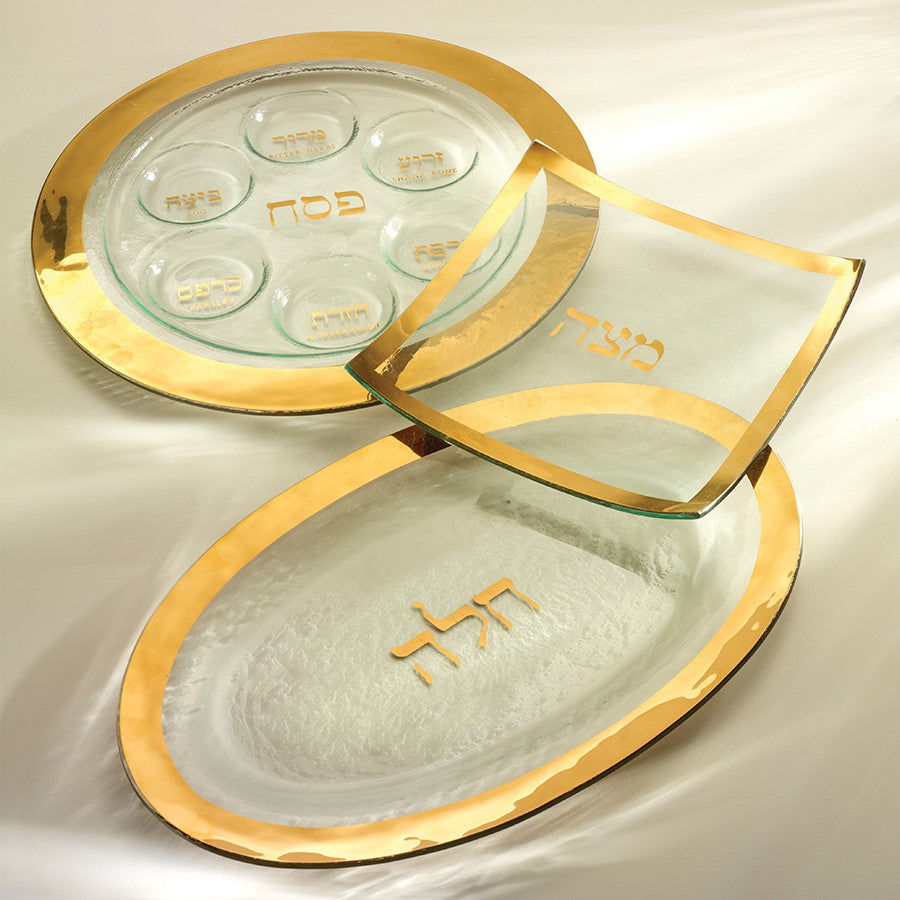In this photograph, we see three intricately designed glass trays, placed on a creamy silk surface. Each tray features a golden rim and Hebrew text in the center, crafted in gold. The tray to the top left is circular, adorned with six round indentations, each containing golden Hebrew text. The tray on the right is almost square with curved corners and golden Hebrew inscriptions in the middle. The smallest tray, positioned at the bottom, is elliptical and also showcases Hebrew text in its center. The background is grey with interplay of shadows and light, adding depth to the elegant presentation of these traditional Jewish dishes.